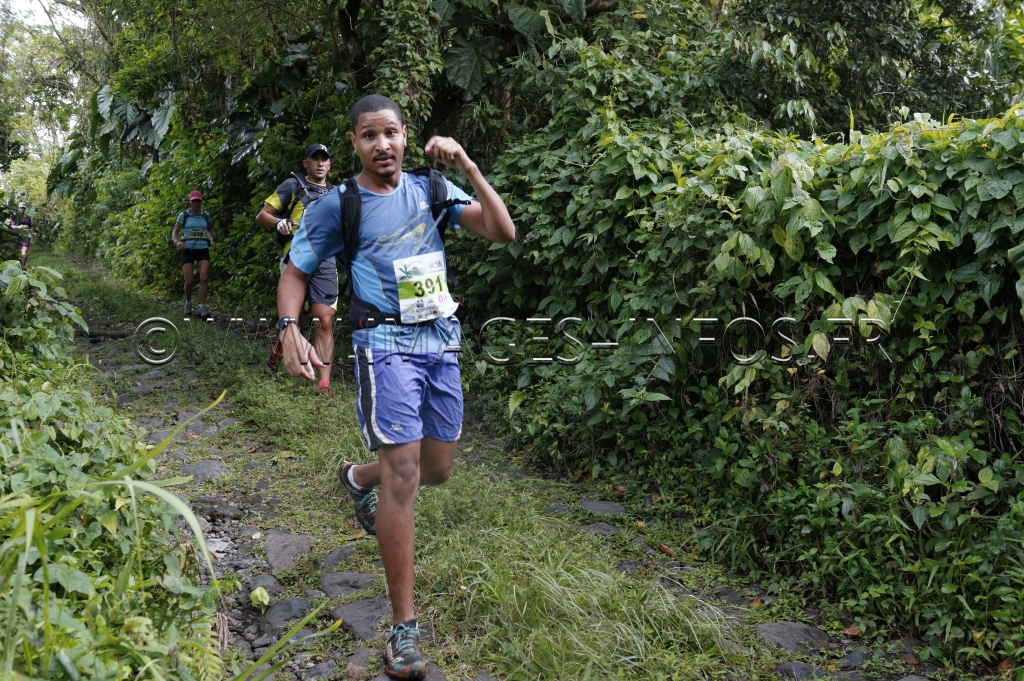This photograph captures a trail running race set in a lush, jungle-like environment with thick green vines, palm trees, and dense vegetation bordering a muddy, rock-strewn path, which vehicles have clearly traversed, indicated by a central strip of grass. Prominently watermarked with a copyright symbol and the URL www.images.info.fr, the image features three athletes navigating the terrain. Leading the pack is a tall, black man with short-cropped hair, a mustache, and a sports watch, dressed in a blue shirt and long blue shorts adorned with a blue and white stripe. His race bib, numbered 391, is visible as he looks directly at the camera with his left arm bent at the elbow. Following him is a Caucasian man partly obscured by the leader's arm, distinguished by his orange or red shoes and gray shorts. The third runner, potentially a female, wears a tealish blue shirt, a pinkish hat, shorter black shorts, and running shoes. Notably, all three runners appear to be carrying backpacks, underscoring the race's challenging nature through this verdant, tropical setting.